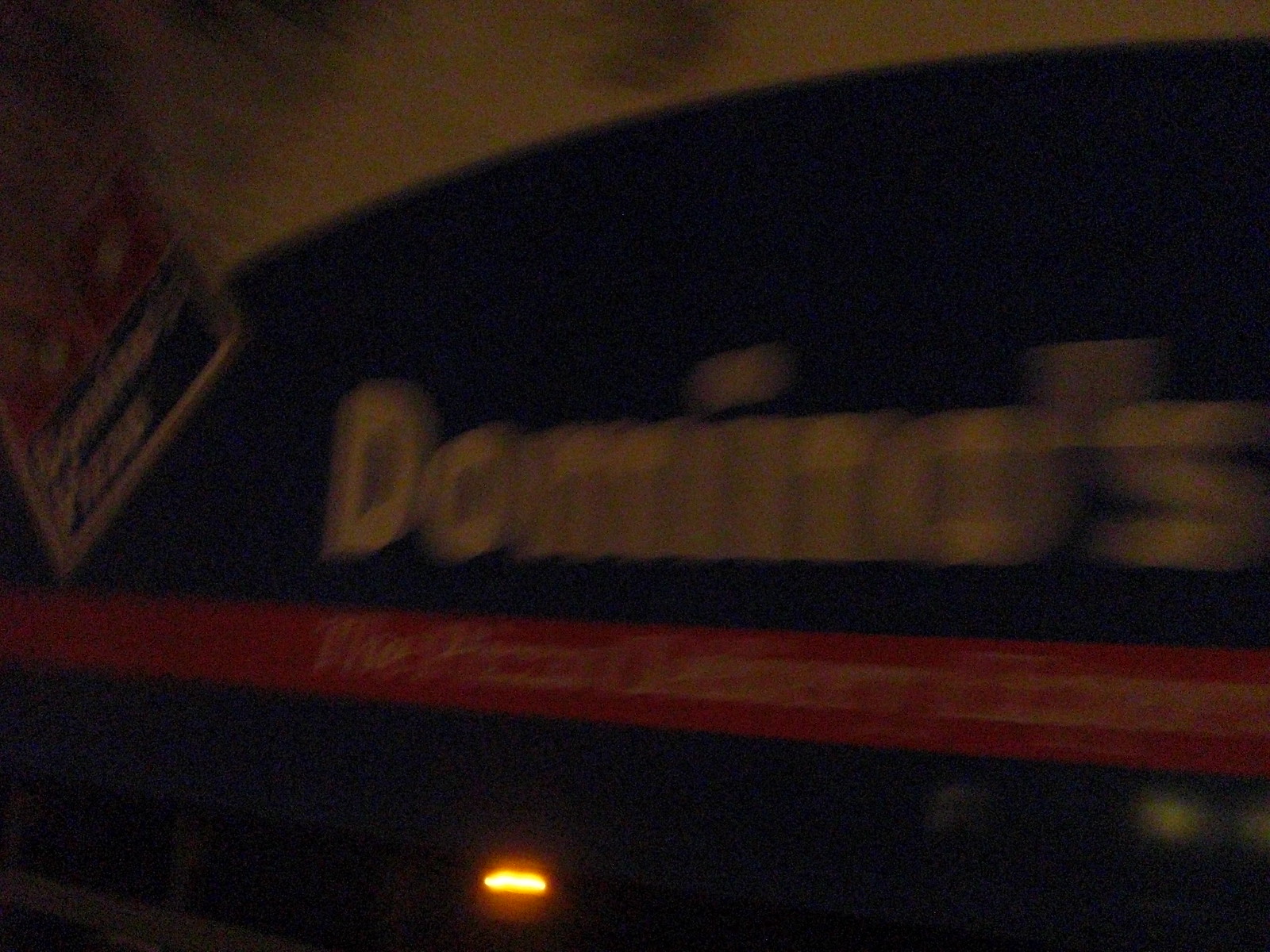A partial view of a Domino's sign is visible in this image, with the recognizable "Domino's" text displayed prominently in white font against a blue background. Below the text, there is a red banner, also with white font, but the words are too blurry to decipher. On the left side of the sign, the iconic red Domino's logo can be seen, partially emerging from behind the sign. The photograph appears to have been taken at night, resulting in a dark and grainy quality that obscures finer details. Overall, the scene gives an impression of a dimly lit area with limited visibility.